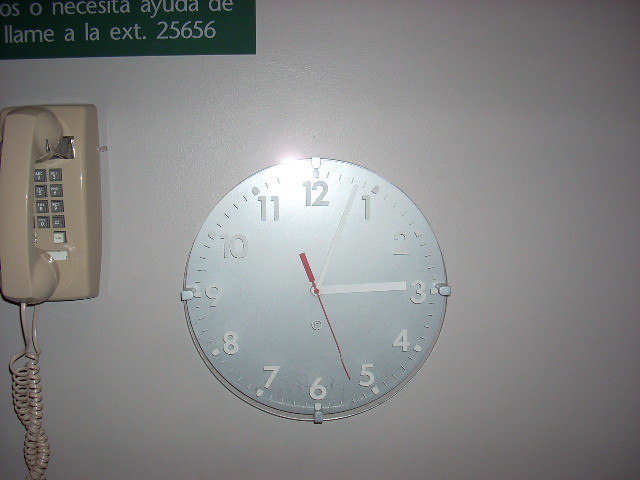This color photograph features a round, silver wall clock set against a greyish wall. The clock face displays white numerals from one to twelve, interspersed with small black or possibly silver markers, and accented by tiny white dots positioned just outside the numerals. The clock's hands are white, and the time shown is approximately five past three. Additionally, a red second hand points just below the five. 

To the left of the clock, a cream-colored telephone, reminiscent of an 80s style, hangs on the wall. The telephone features a keypad with black square buttons marked with white characters. A coiled cord hangs from the phone, and the handset rests in its cradle. Above the telephone, a greenish sign with white writing is visible; the text is not in English but includes the number 25656 located at the upper left corner of the sign.